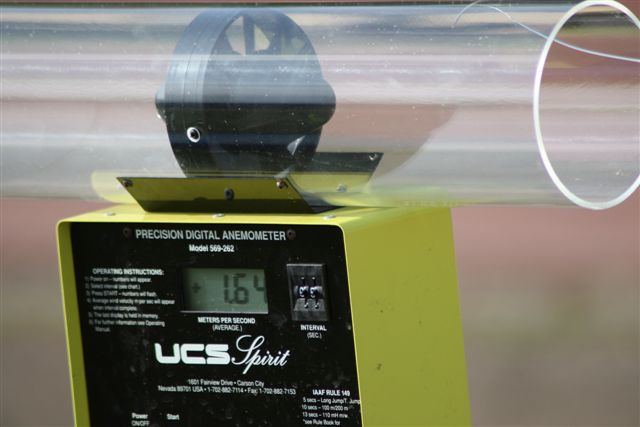This horizontal, rectangular photograph showcases a large, precision digital anemometer machine. The machine features a light yellow outer casing with a black front panel adorned with white lettering. At the top of the front panel, "Precision Digital Anemometer" is prominently displayed, followed by the model number and "USC Spirit" beneath it. On the left side of the machine, operating instructions are clearly visible. Central to the machine's face is a screen that displays the measurement "1.64". On the right side, there are a couple of metal switches that add to the machine's intricate design. Atop the machine sits a large black wheel, resting on a piece of curved silver metal. The background of the photograph is intentionally blurred, creating an out-of-focus effect with colors predominantly in pink, black, and gray. Notably, a large white oval is positioned in the upper right-hand corner, adding a distinctive element to the composition.